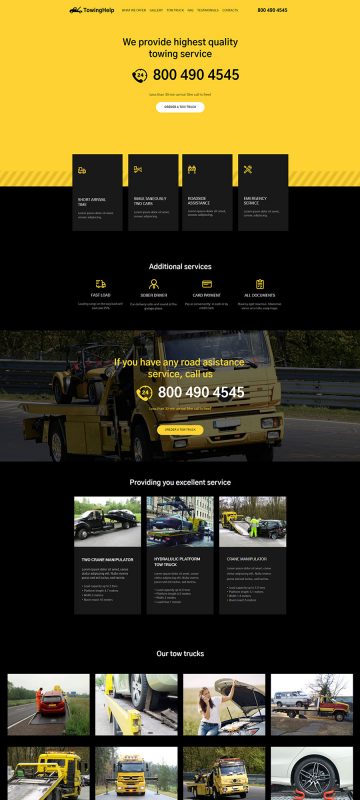The image is a detailed capture of a towing service website. At the top, the header features a gold background with black font, including a black car icon, navigation menus, and a phone number (1-800-490-4545) beside a phone icon with "24". The header text reads, "We provide the highest quality towing service". Below this, a prominent black sentence is displayed followed by a white text box outlined in black.

Next, the website showcases four black squares each containing gold icons and white text, too small to discern. Further down, the section titled "Additional Services" features four more gold icons with corresponding white text.

An image below this section depicts a yellow tow truck on a street, surrounded by green trees. A gold text box states, "If you have any road assistance service, call us 1-800-490-4545". Moving along, three images are displayed: 
1. A black tow truck towing a black car.
2. A gold tow truck towing a dark-colored vehicle in a city setting.
3. A person in green standing beside a dark vehicle and a tow truck.

Further down, there's a section titled "Our New Trucks" in white font, featuring a series of images:
1. A person in orange beside a red car on a tow truck.
2. A car on a street.
3. A woman in white and jeans sitting by the hood of her car with the hood up.
4. A red tow truck with a white vehicle.
5. Another view of a yellow tow truck.
6. A yellow tow truck.
7. A yellow tow truck again.
8. A white vehicle with a black wheel and a red object near the wheel.